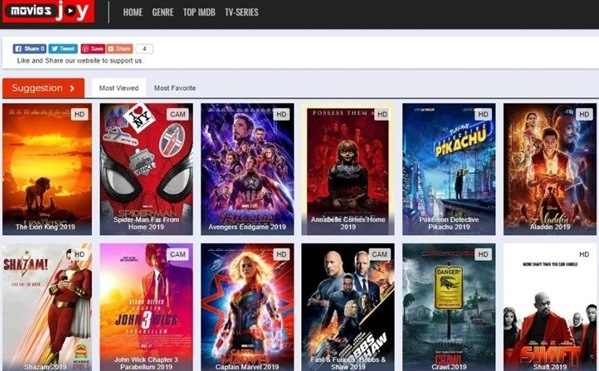The image showcases a prominent movie streaming website named MoviesJoy, identifiable by its label in the top left-hand corner. This platform provides users the opportunity to watch a variety of films for free. The homepage features numerous movie titles, including popular ones like "The Avengers: Endgame," "Annabelle," "Aladdin," "Shaft," "Captain Marvel," "John Wick 3," "Spider-Man: Far From Home," and "Pokemon Detective Pikachu" (2019). The website's navigation bar, positioned at the top right, offers several sections: Home, Genre, Top, IMDB, and TV Series, allowing users to explore different categories and selections.